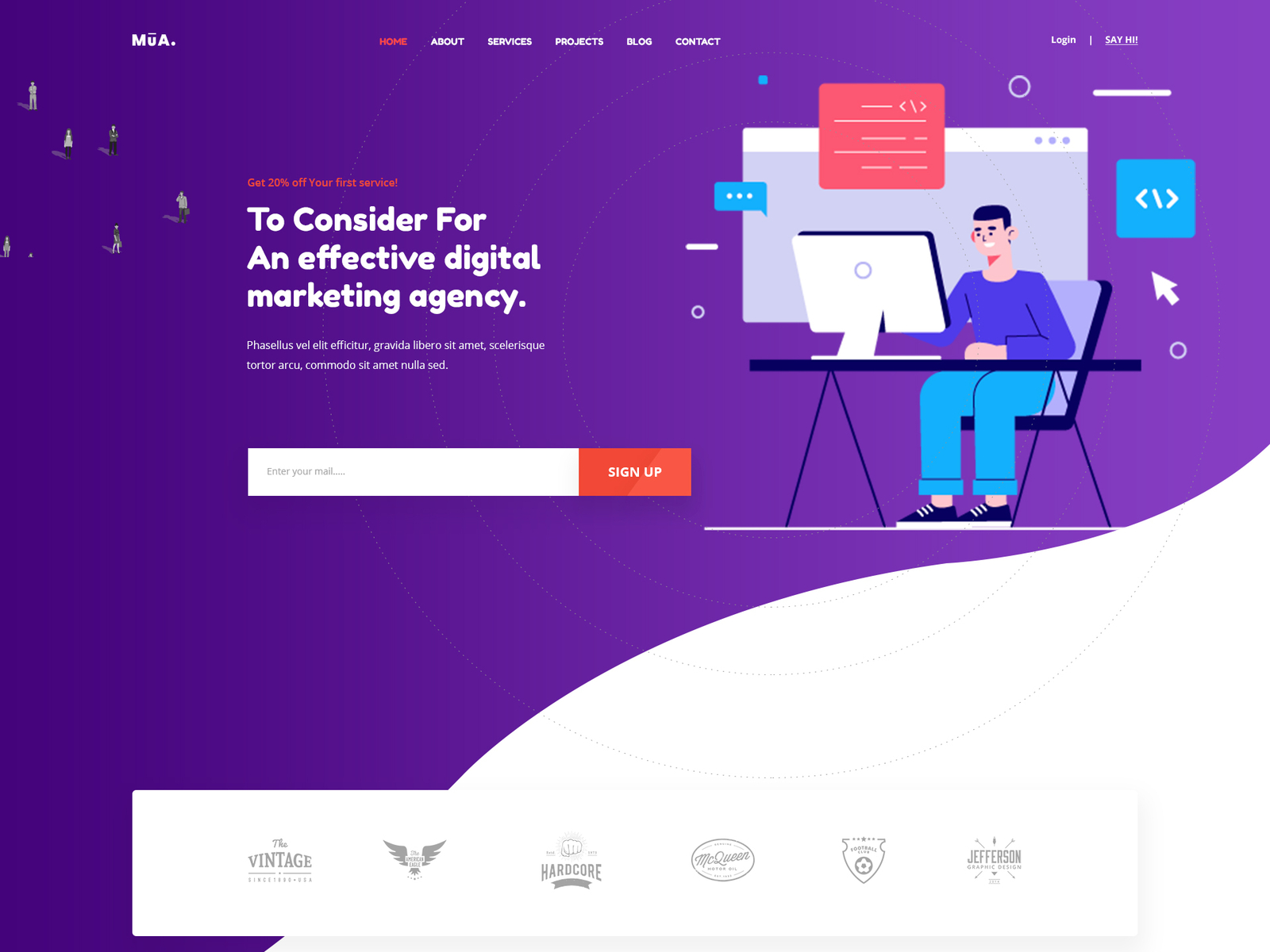Website Homepage: MULA

The homepage of the website, branded as **MULA.**, showcases its name prominently with a line above the 'U'. Both the 'M' and 'A' are capitalized, contributing to the modern and clean aesthetic. The dot at the end of the name adds a unique touch to the branding.

The top navigation bar features several tabs: Home, Belt, Services, Projects, Blog, and Contact. The 'Home' tab is highlighted in red, indicating the current page. The background of the page is a rich, eye-catching purple.

On the right side of the homepage, there is a minimalist illustration of a man sitting at a desk with simple depictions of a computer setup behind him, evoking a modern workspace theme. To the left of this illustration, a prominent banner reads "Get 20% off your first service," accompanied by another message about the keys to effective visual marketing. This section emphasizes promotional offers and insights into their marketing strategies.

Below this banner, placeholder text in Latin (likely Lorem Ipsum) occupies a box, suggesting additional information or content to be updated. Adjacent to this box is a noticeable 'Sign Up' button, inviting users to register.

Overall, the design is streamlined with a focus on user engagement and easy navigation.